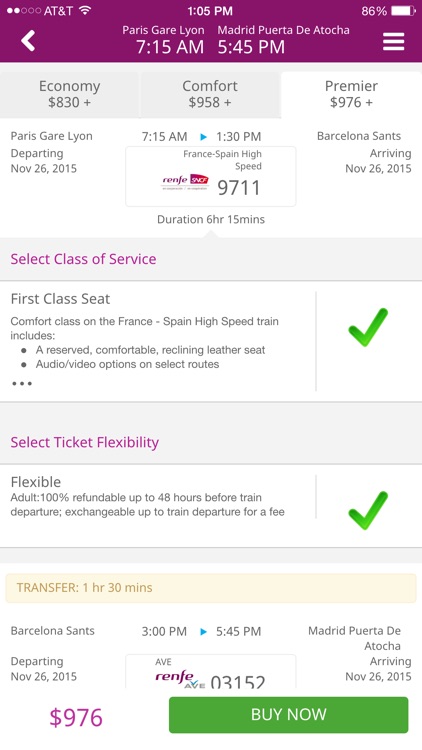The screenshot displays a transportation booking interface. The header at the top of the image is in a plum color. In the upper left corner, there are indicators showing two out of five bars for AT&T reception and a lit Wi-Fi icon. The center of the header displays the time as 1:05 p.m., and the upper right corner shows a battery icon with an 86% charge.

Below the header, the main content is divided into several sections. The first line reads "Paris-Guerre-Lyon" followed by the time "7:15 a.m." To the right of this text, another line reads "Madrid-Porto de Otocha 5:45 p.m."

Under these details, a white background section spans the width of the screen, featuring three buttons aligned horizontally. From left to right, the buttons are labeled:
- "Economy $830"
- "Comfort $958"
- "Premier $976 and up"

Below these buttons, in purple text, the instructions "Select class of service." are provided. Supplementing this, there is a descriptive text explaining that the "First class seat comfort class on the France-Spain high-speed train includes a reserved, comfortable, reclining leather seat," accompanied by a green checkmark to the right, indicating confirmation or selection.

At the bottom-right corner of the image, there is a large green button with light green text that reads "Buy Now."